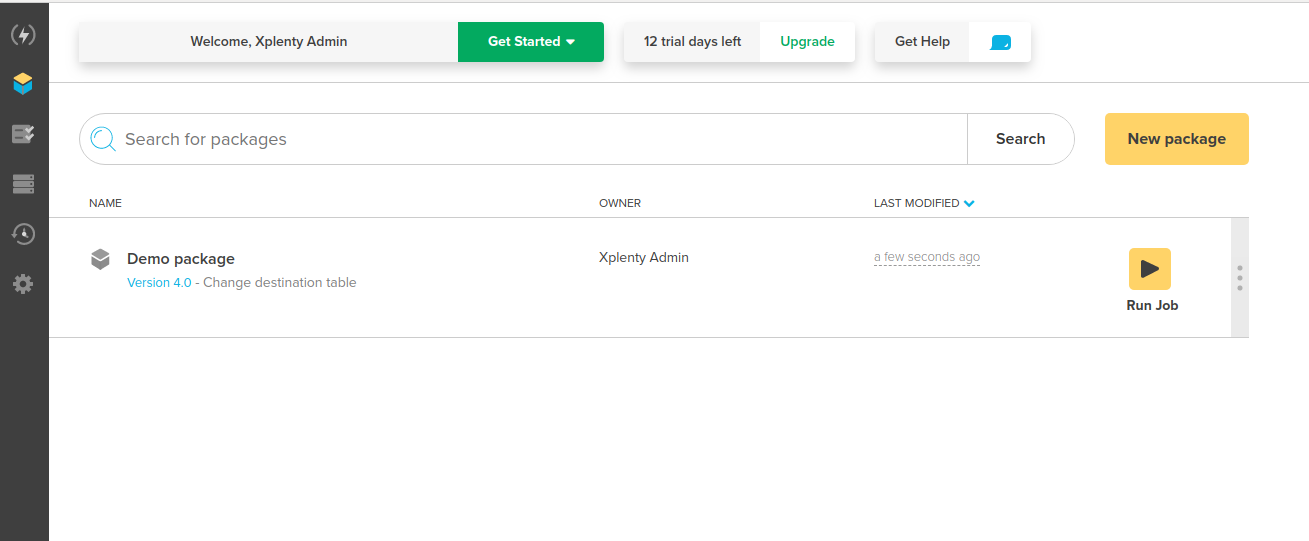This image is a horizontal screenshot of a web interface displayed on a white background. On the left side of the screen, there is a dark grey vertical toolbar featuring six icons. The second icon from the top is highlighted, depicting a three-dimensional square with blue sides and a yellow top. 

At the top of the main interface, a header bar contains a white box with the text "Welcome Xplenty Admin." Adjacent to this is a green "Get Started" dropdown button. To the right, another box displays "12 Trial Days Left," accompanied by a green "Upgrade" text button and a "Get Help" button featuring a blue message icon.

Below the header, there's a long search bar labeled "Search for Packages," adorned with a blue magnifying glass icon on the left and a search link on the right. To the right of the search bar, a yellowish-orange button is labeled "New Package."

The main content area lists available packages, displaying columns for the name, owner, and last modification details. The highlighted package is "Demo Package version 4.0," with "version 4.0" appearing as a blue hyperlink. The owner is "Xplenty Admin," and the last modification was "a few seconds ago."

To the right of this listing, there is a small orange-yellow button with a black triangle labeled "Run Job," which is used to execute the demo package.